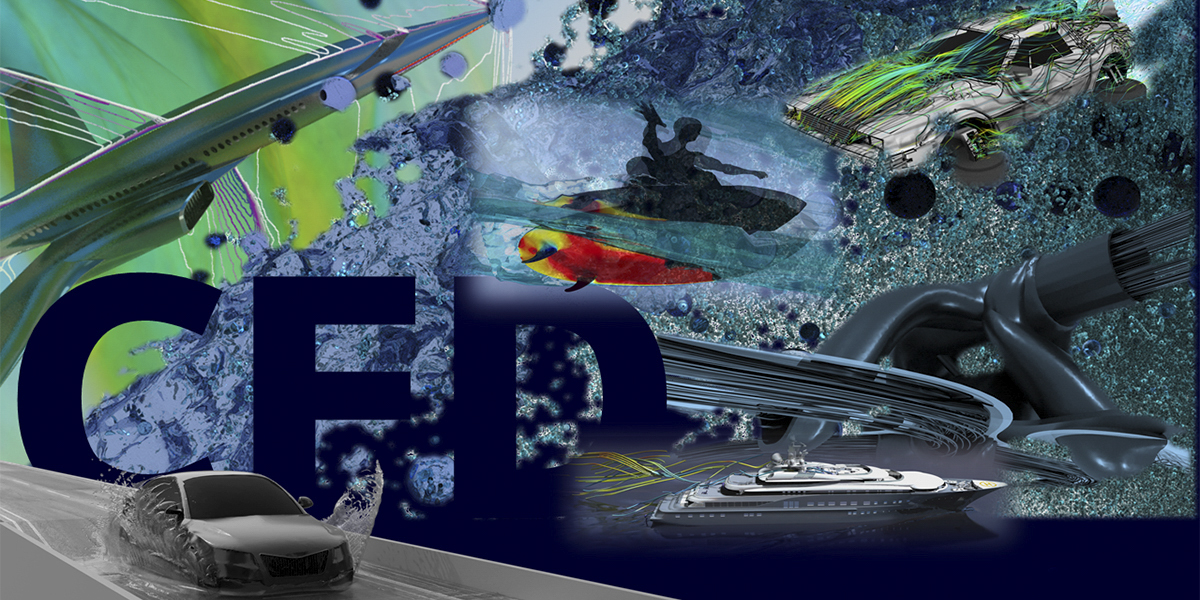The image is an abstract artwork featuring a dynamic collage of various shapes and objects. Dominated by a gray asphalt road, a speeding gray car creates dramatic splashes of water around it. In the upper left corner, a model plane appears against a green backdrop with the blue letters "CED" (or possibly "CFD") behind it. A mystical rock or crystal and a figure casting their hands out are placed centrally, adding an enigmatic touch. The bottom right shows a cartoony cruise ship on a blue background, while the top right features a truck intricately covered in rainbow-colored wires, resembling a hover car. The background is a vibrant mix of colors, including black, white, gray, brown, yellow, blue, dark blue, teal, purple, yellow, and red, possibly portrayed as glitter or scattered paint, enhancing the mosaic's complexity. The only text visible reads "CED" in bold blue letters, though there's a slight ambiguity about it being "CFD."